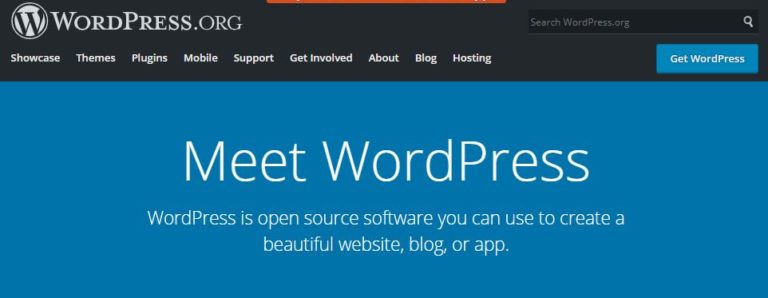The image showcases a webpage with a prominent black border at the top. In the top left corner, there is a white circle featuring a black "W" in the center, surrounded by a thin black ring. Next to this, in large white capital letters, it reads "WordPress.org." 

Positioned centrally at the very top of the image, a thin orange line runs horizontally. On the right side of the header, there is a search bar displaying the text, "Search WordPress.org," accompanied by a magnifying glass icon.

Below the search bar, there is a navigational menu with clickable options including: Showcase, Themes, Plugins, Mobile, Support, Get Involved, About, Blog, Hosting. 

To the right of the menu, there is a small rectangular blue button that says "Get WordPress."

Beneath this section, the background turns dark blue. In large, bold white letters, it reads, "Meet WordPress." Below that, in smaller, regular white letters, the text states: "WordPress is open source software that you can use to create a beautiful website, blog, or app."